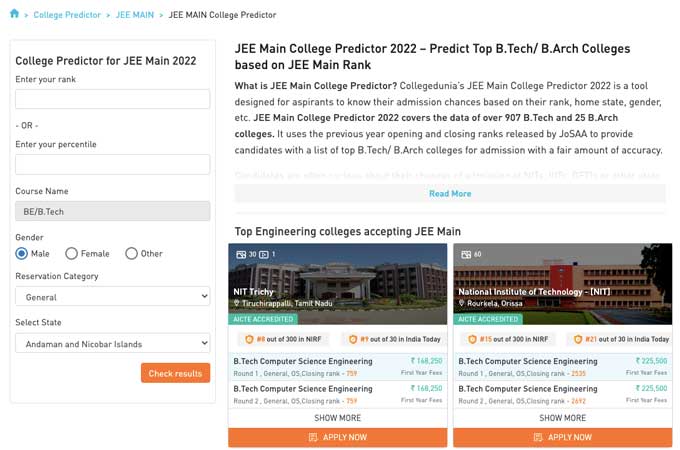The image depicts a webpage dedicated to a College Predictor tool specifically for JEE Main 2022 aspirants. At the top, the header prominently displays "College Predictor, GMAIN, GMAIN College Predictor" in a striking manner. The top-left corner of the page shows the navigation path in blue text.

On the left side of the webpage, a main icon labeled "College Predictor for JEE, May 2022" captures attention. Below this, there are input fields for users to enter their rank or percentile. Additionally, dropdown options allow users to select their course (BE or B.Tech), gender (male, female, or other), and reservation category (general). Another dropdown is provided to select the state, but intriguingly, one of the options mentioned is "Nicole Islands." At the bottom of this section, there's a prominent orange button labeled "Check Result."

The right side of the page starts with a black text that reads "JEE May 2022 predicts top B.Tech/B.Arch Colleges based on JEE Main rank." Below this, a detailed description reads, "What is JEE Main College Predictor? JEE Main College Predictor 2022 is a tool designed for aspirants to know their admission chances based on their rank, home state, gender. The JEE Main College Predictor 2022 covers data from over 970 B.Tech and 25 B.Arch colleges. It uses the previous year's opening and closing rank released by JOSAA to provide candidates with a list of top B.Tech/B.Arch colleges for admissions with a fair amount of accuracy." At the bottom of this text, a blue "read more" link invites further exploration.

At the bottom of the webpage, there is a section titled "Top Engineering Colleges Accepting JEE Main." Listed here are colleges such as NIT (National Institute of Technology), though the text appears slightly blurry. Each college listing includes an orange "Apply Now" button encouraging users to initiate their application process.